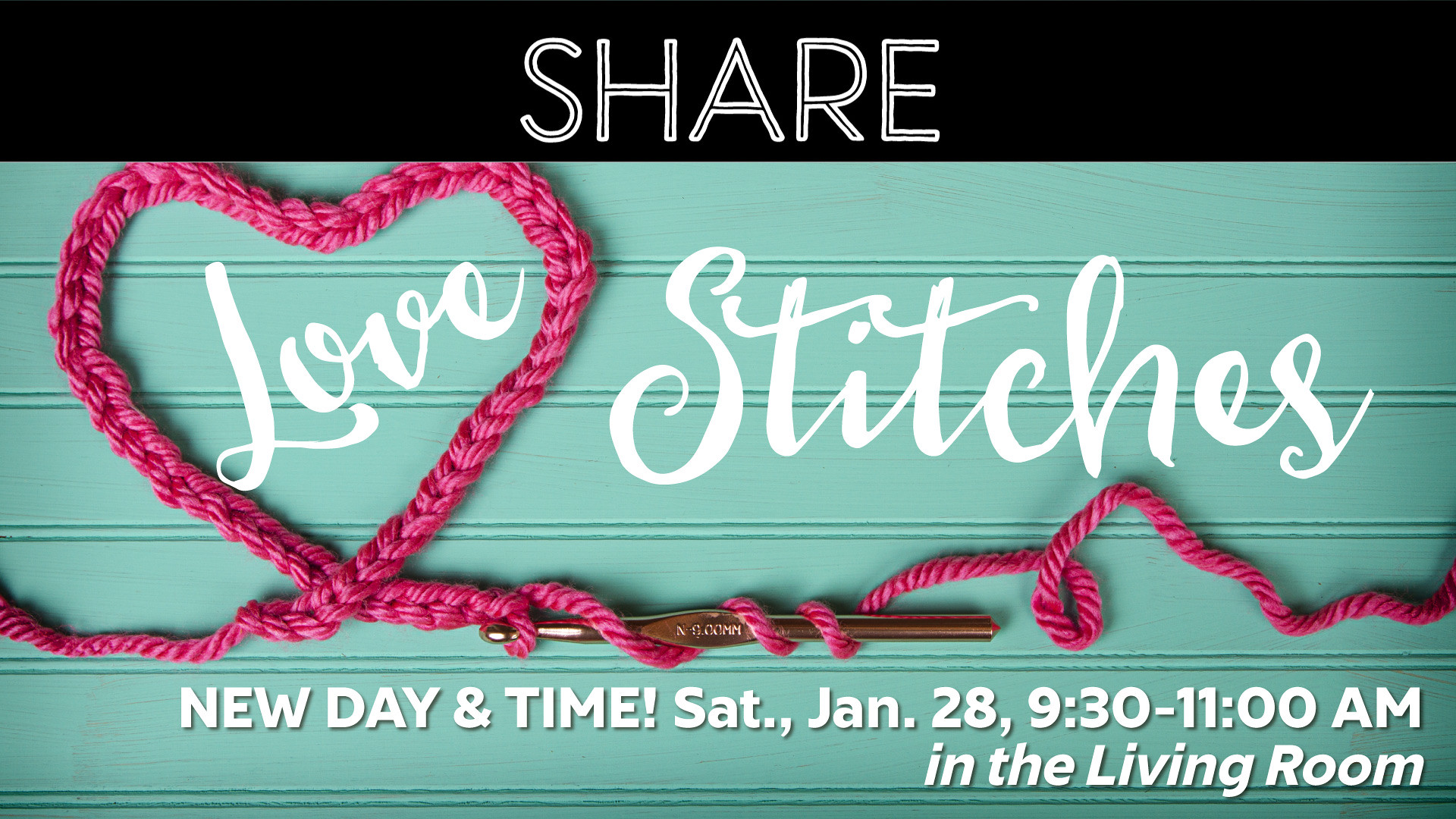This image is a flyer advertising an event called "Share Love Stitches," scheduled for Saturday, January 28th, from 9:30 to 11 AM in the living room. The top of the flyer features a long black rectangle with the word "SHARE" in bold, white, capital letters. Below this, a cord, resembling a crochet or shoelace, forms a heart shape and is intricately wrapped around a copper-colored crochet hook. Inside the heart, the word "LOVE" is written in white cursive, while "STITCHES" is positioned to the right, also in cursive. Scattered red hearts adorn the image, which is set against an aquamarine wooden background with lines suggesting a painted table or paneled wall. The bottom section of the flyer prominently displays the new date and time details in white text, emphasizing a creative and inviting design that invites people to join a stitching or knitting session.